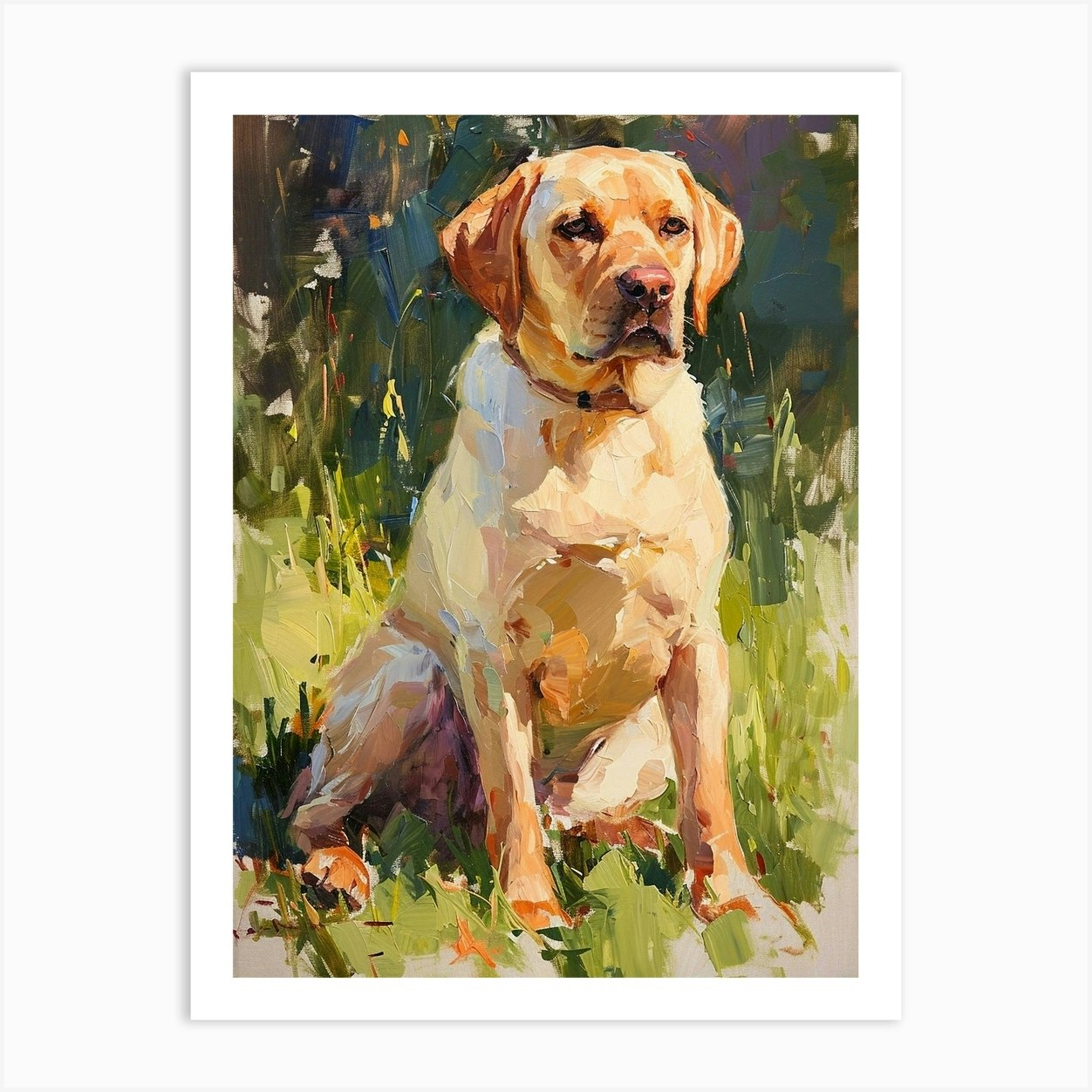The image displays a detailed, hand-painted oil or acrylic painting of a large, beige-colored dog, reminiscent of a golden retriever or yellow lab, sitting on its haunches with its front legs poised in front. The dog's fur has hints of golden and orange, particularly noticeable on its face, ears, lower legs, and paws. Its eyes are amber, and a small pink nose adds a touch of character. The dog wears a brown collar and is positioned in a lush green field, surrounded by various shades of green grass and dark evergreen trees in the background. The artwork is encased in a white frame. A small orange element is visible in the bottom left-hand corner, potentially part of the dog's body or another object. Overall, the painting beautifully captures the lifelike essence of the dog, giving the impression of an alive, soulful presence.